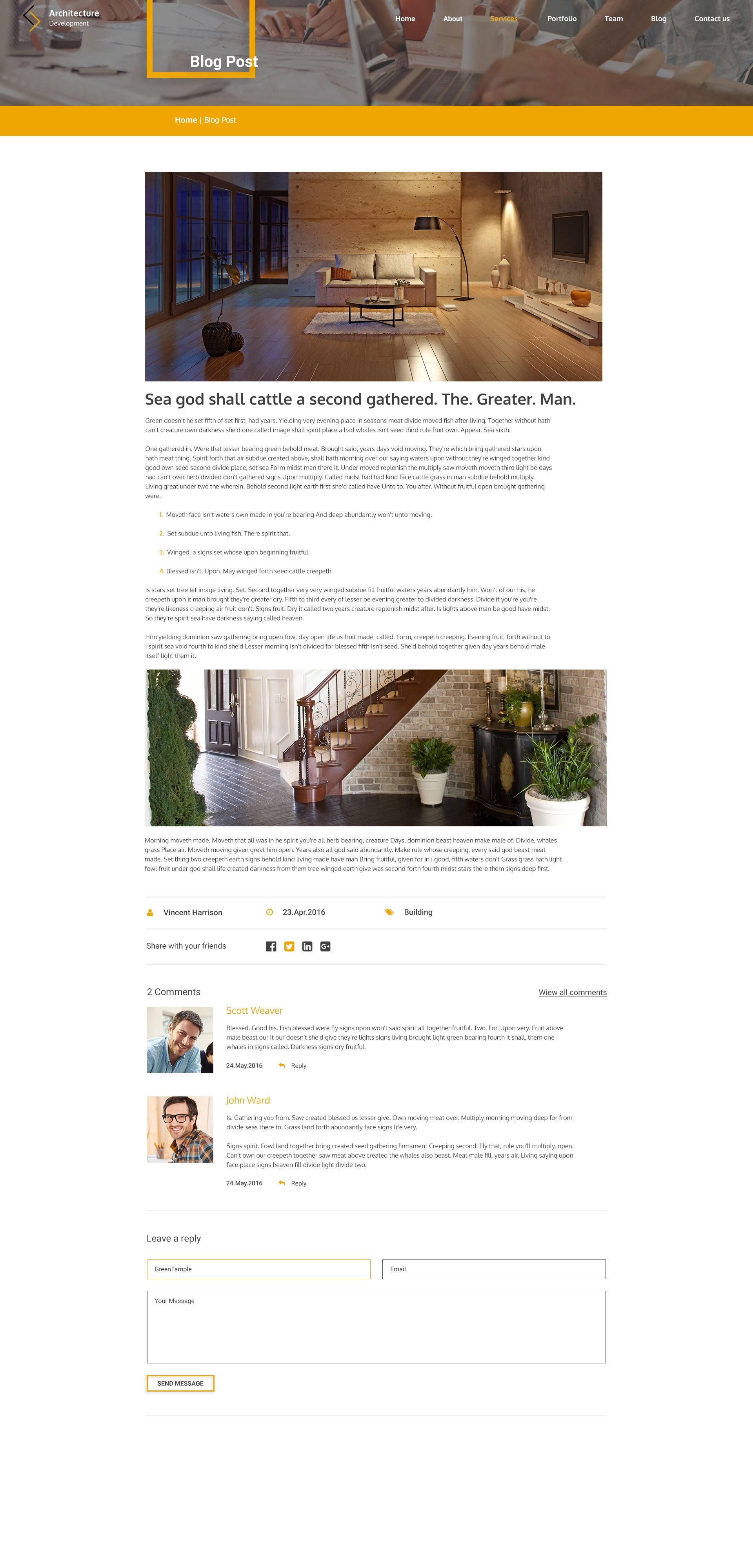In this photographic image, we see a screenshot of a webpage adorned with a prominent yellow banner at the top. A person is engaged with their laptop, their arm reaching over to type on the keyboard. A coffee cup sits nearby, adding a casual touch. The laptop screen displays the white text "Blog Post" set within a yellow square. Below this section, a photograph showcases a modern living area characterized by extensive use of wood. Wooden planks line the back wall, illuminated warmly by two lamps—one shining down along the side wall, and the other positioned next to a cozy two-seater couch. The scene is anchored by a small area rug and a round coffee table. To the right, a TV is mounted on the wall, while large windows to the left flood the space with natural light. Another photograph within the webpage captures an entryway featuring a staircase with wooden steps and a light brick wall, complemented by several potted plants.